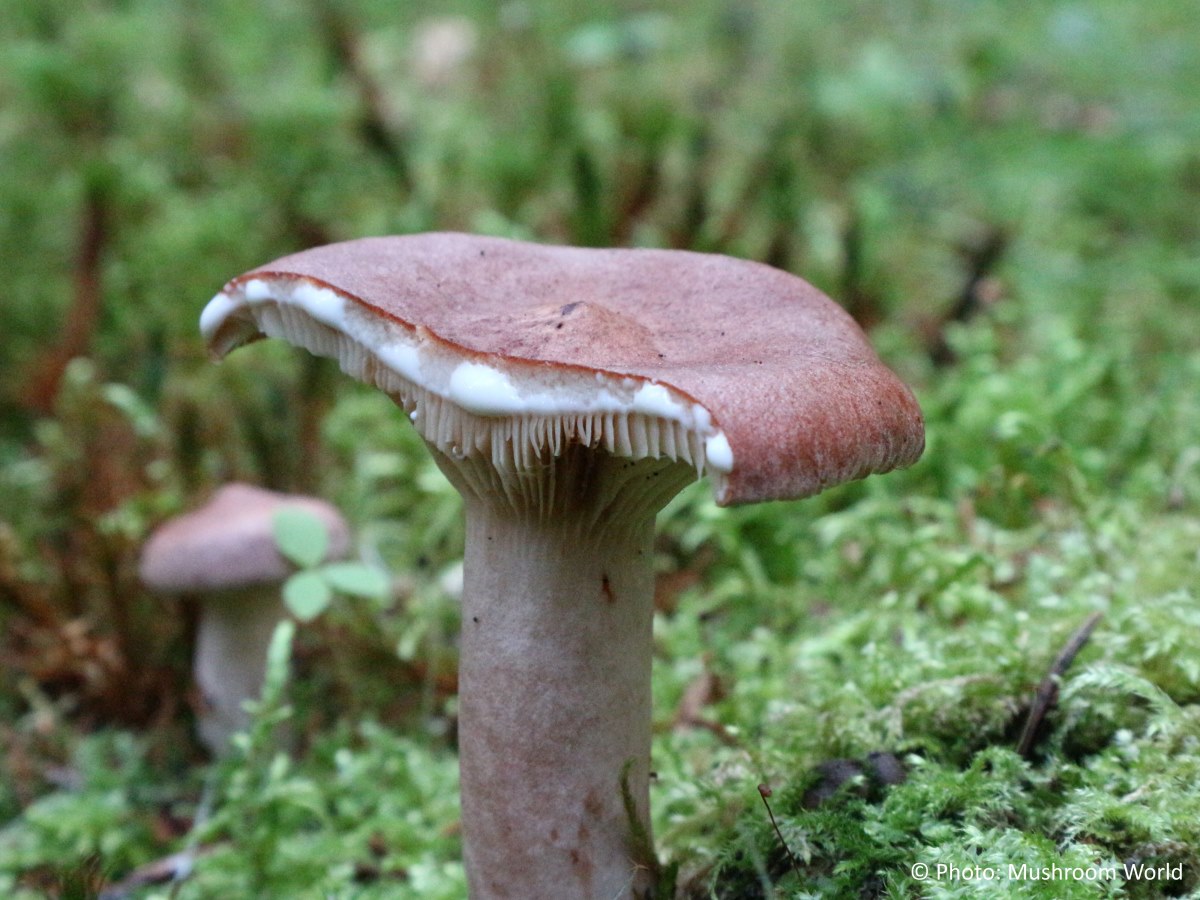This outdoor photograph features a prominently displayed mushroom situated amidst a bed of grass and light green foliage. The central mushroom, dominating two-thirds of the image height, has a tan-gray stalk and a reddish-brown cap that appears to have been cleanly split in half. The exposed section reveals a white, fibrous interior with what looks like milky white liquid oozing out. The backdrop of the image is a blurred mix of leaves, branches, and grass, emphasizing the mushroom's focus. In the bottom left corner, there's a smaller, intact mushroom of the same variety with a similar reddish-brown cap and light gray stalk. Notably, the bottom right corner of the image bears a "Photo Mushroom World" copyright mark in white. The setting exudes a damp, natural environment, enhanced by the slightly blurred greenery and moss that frame the scene.